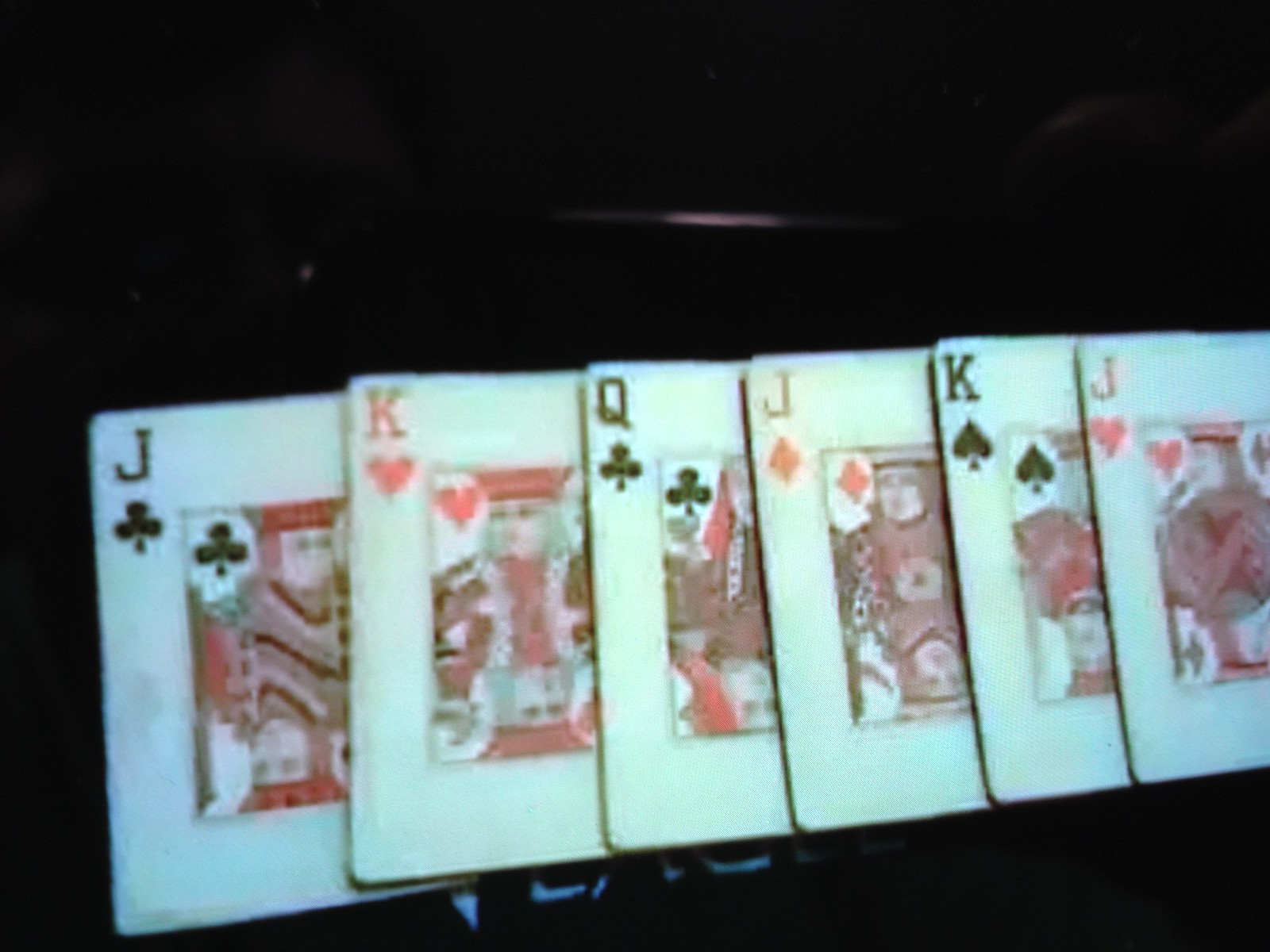This is a photograph of a pixelated screen, capturing a series of face cards from a deck of playing cards. The cards depicted are, from left to right: Jack of Spades, King of Hearts, Queen of Spades, Jack of Clubs, Queen of Clubs, Jack of Diamonds, King of Spades, and Jack of Hearts. The background of the photograph is black, accentuating the primary colors of the cards, which are black, white, red, and gray. The cards are arranged in an overlapping sequence, with the bottom-most card starting on the far left and the uppermost card ending on the far right. Due to the blurriness, it is evident that the image is a photo of a screen rather than the actual physical cards.